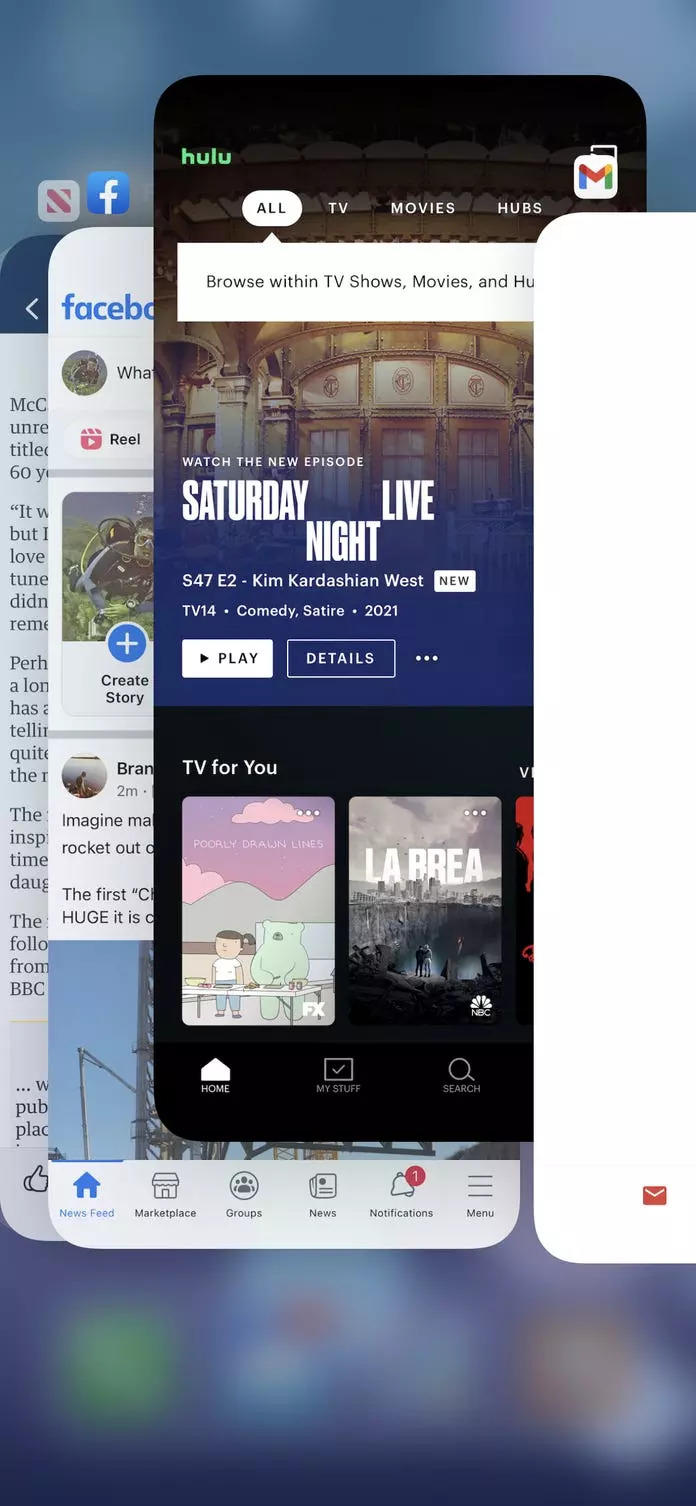A vertically oriented image showcases a smartphone’s home screen with a purple background, upon which various blurred-out app icons are subtly visible. Dominating the foreground are multiple overlapping app screens. 

The foremost screen is partially visible and entirely white, adorned with a red email envelope icon in the bottom left corner. Just behind it lies a screen with a black background displaying the Hulu app. On this Hulu interface, the Hulu logo appears in green at the upper left, followed by the sections "All," "TV," "Movies," and "Hubs." The "All" section is selected. Below this section, a white ribbon reads, "Browse within TV shows, movies, and Hulu." Highlighted beneath is a feature for "Saturday Night Live, Season 47, Episode 2, Kim Kardashian West," with options to either play the episode or view details. Further down, white text on a black background reads "TV for you," listing several recommended shows in rectangular thumbnails.

Continuing into the depth of the layered apps, a screen displaying Facebook is partly visible. The layout suggests it’s on the homepage of a user’s profile, showing the user’s profile picture and the phrase "What's on your mind?" commonly found at the top of Facebook’s homepage. The final discernible layer is a page featuring a black banner on top, filled with extensive text that resembles content from an e-book or an online article. The exact text is illegible, hinting that it is part of a book or an article being read or listened to.

This image captures the vibrant and busy nature of a smartphone’s active interface, with multiple apps opened and layered over a subtly hued background.